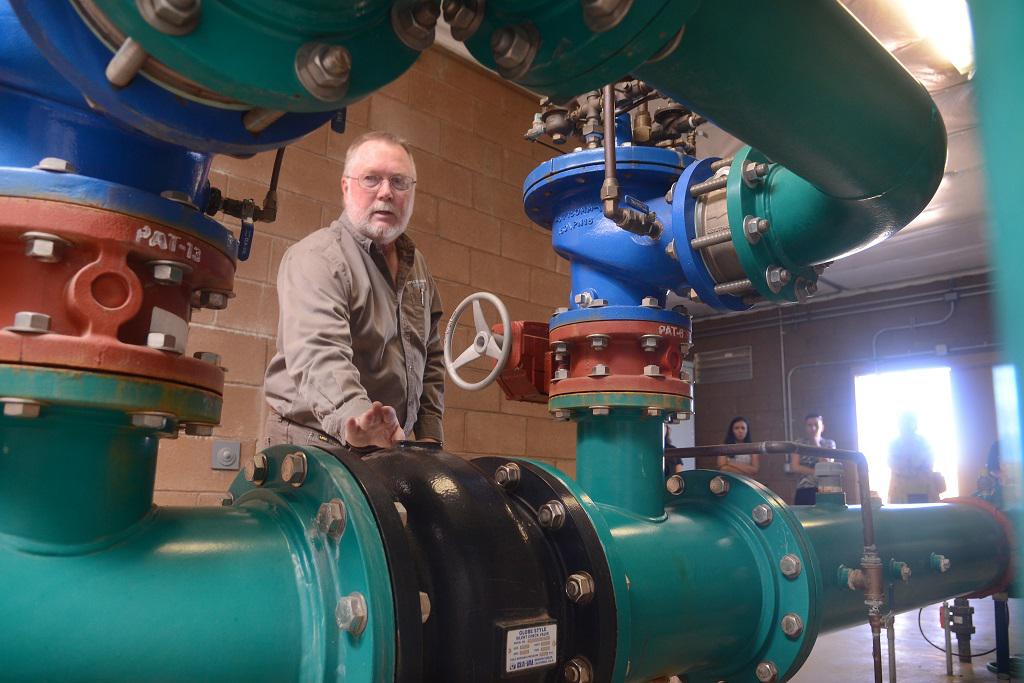In the photograph, a Caucasian man with a white beard and a brown button-down collar shirt stands amidst an intricate network of large, colorful pipes. These pipes, bolted together, come in shades of green, black, red, and blue, with some transitioning between colors at various connection points. A prominent green pipe runs horizontally, morphing into black in the center, before reverting to green. Above it, a cylindrical red pipe connects to a blue segment, while copper pipes branch out from the blue sections. Beside the man, there's a valve wheel for controlling the flow within the pipes.

The man stands with his right arm extended outward and his palm facing up, observing the pipes. To the right side of the image, a group of people watches him, backlit by bright white light streaming through a large window. Behind these onlookers, thin metallic pipes are visible, crisscrossing along a stone wall. The sunlight illuminates the scene, highlighting the interconnected industrial setup and the attentive audience.